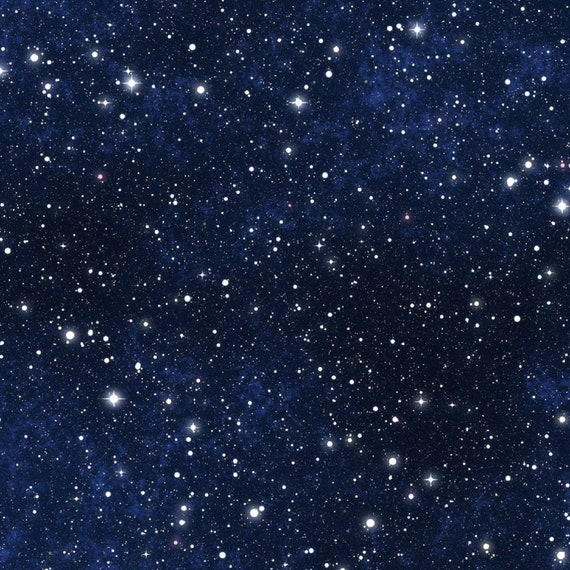This nighttime image captures a vast, star-studded sky, predominantly painted in deep blues and blacks. The celestial display features numerous vibrant stars, some of which could be planets, scattered across the sky. These stars vary in shape, with many appearing as bright circles while others resemble diamonds, each surrounded by a lighter, white aura. The sky's color transitions, with more blue dominating the left upper and bottom corners, and the right upper corner, while the blackness seems to dip downwards from the middle to the bottom right. Among the stars, a few exhibit distinct light rays extending horizontally and vertically, adding a sense of depth. Additionally, a faint, bluish-gray fog or gas drifts across the scene, primarily from the bottom right toward the middle, enhancing the outer space aesthetic. Although constellations are not clearly identified, there’s a hint that the bottom left might form the Big Dipper. The scene has a science fiction quality, with the all-black background and the numerous, twinkling, variably-sized stars, suggesting it might be a computer-generated graphic.